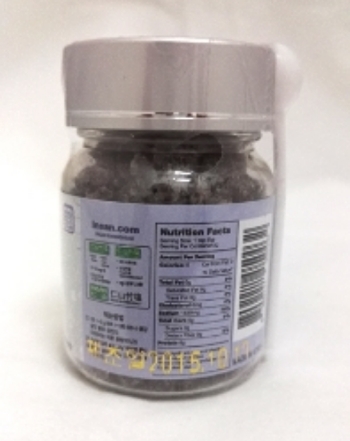The image captures a close-up of a small, vertically aligned, slightly rectangular bottle. The bottle is short, round, and made of clear material, with a silver lid. Attached vertically to the right side of the bottle is a tiny white measuring scoop, with the scoop part positioned against the lid and the handle extending down along the bottle's side. The bottle features a purple label that appears blurry, although the nutritional facts box is somewhat discernible. Above the label, the contents of the bottle are visible through the clear material—showing a very dark, solid-looking substance. At the bottom of the bottle, against the purple label, there is a yellow print, presumably the expiration date, which is also quite blurry.